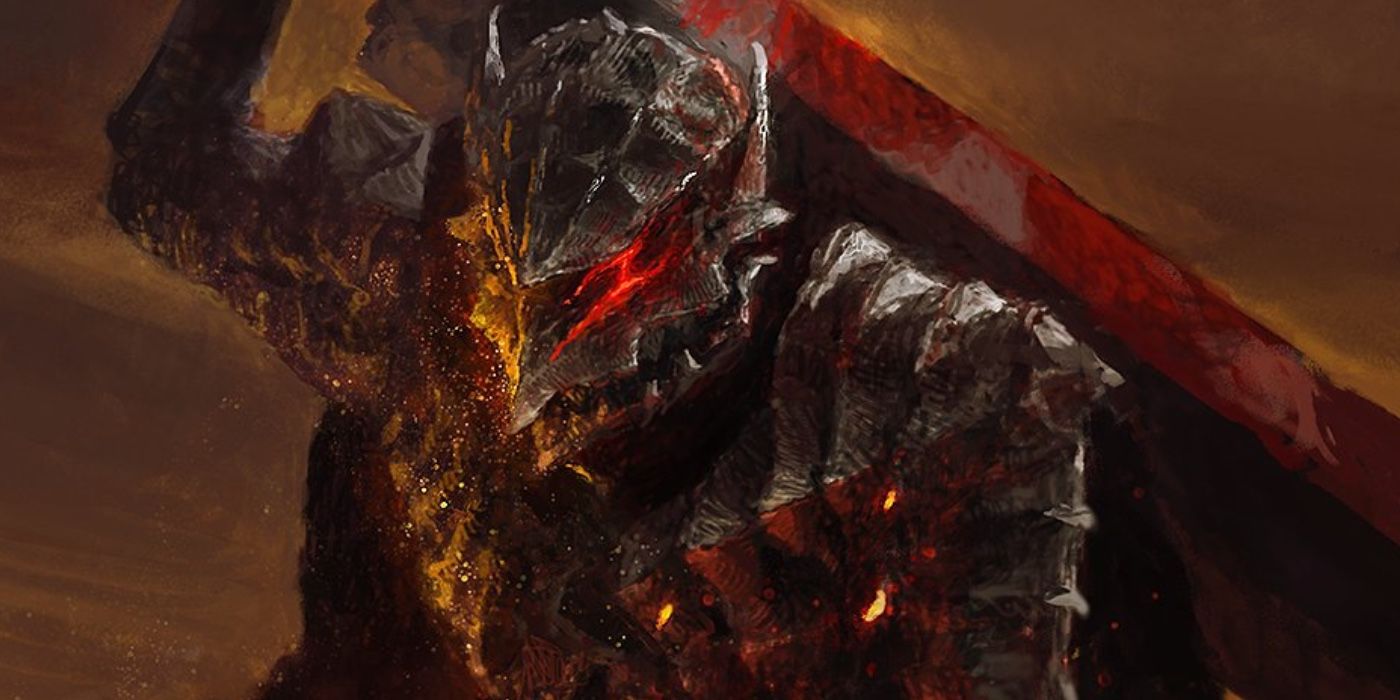The image is a horizontally aligned rectangular artistic piece, likely computer-generated, and potentially depicting a rendition of a character from an anime, possibly Guts. The primary subject is centrally placed, featuring a heavily armored, semi-humanoid figure that resembles a robot or machine. The character appears to be kneeling, with a right arm bent and reaching behind, possibly holding or unsheathing a sword. The armor is predominantly gray with a metallic sheen, and is adorned with pointed tips near the ears. 

The face of the character has a triangular tip and exhibits a mouth and a single glowing red eye, with red, lava-like accents. There is a noticeable amount of gold and brown sparkles emanating from the character. The background is a blur of brown and gray hues, almost like a painted backdrop, without clear borders or defined features, making it challenging to discern whether the setting is indoors or outdoors. 

In the upper right corner, there is a brown triangle, which some perceive as possibly being a table or counter with a brown top and a thin red strip along its front edge. The overall scene is void of text or any specific indication of the artist, contributing to the abstract and enigmatic nature of the piece.